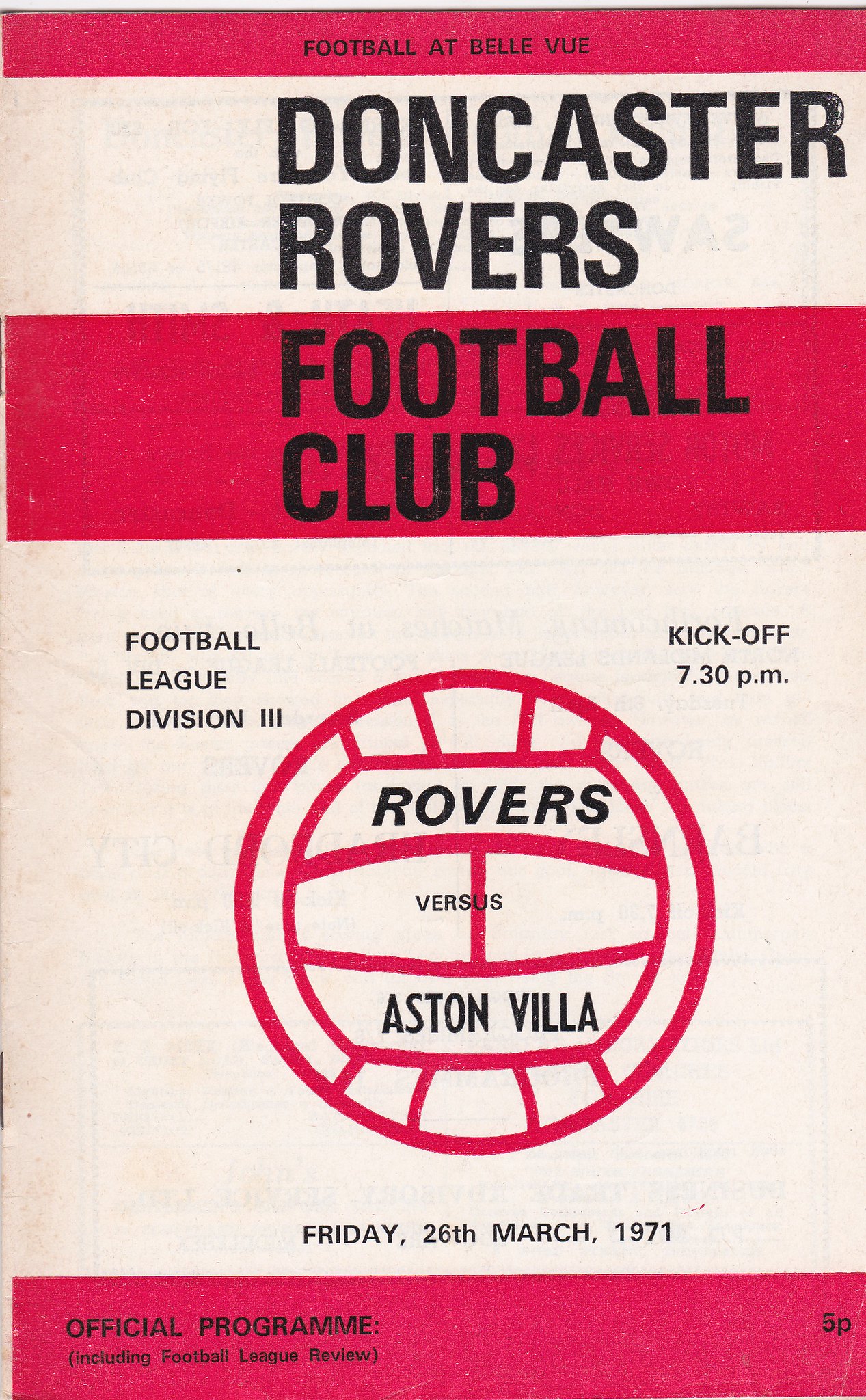This is a photograph of the front cover of an old, worn pamphlet, specifically an official program from a football match at Belle Vue, the home ground of Doncaster Rovers Football Club. The cover features a striking color scheme of red, white, black, and beige. At the very top, there is a thin white and red striped design followed by the heading "Football at Bellevue" in prominent red text. Below this, in large black and white font, it reads "Doncaster Rovers Football Club."

The main section of the cover is beige and includes detailed information about the event. It mentions "Football League Division 3, Kickoff 7:30 p.m." and specifies the teams, "Rovers versus Aston Villa," along with the date, "Friday, 26th March 1971." The centerpiece of this section is a simple, sketched outline of a European football in red. 

At the bottom of the cover is another thick red stripe bearing the text "Official Program including Football League Review," priced at "5p" (five pence). The left side of the pamphlet shows visible staples, indicating how it was bound. Considering its age, the pamphlet has a visually aged and worn appearance, reflective of its over 50 years of history.